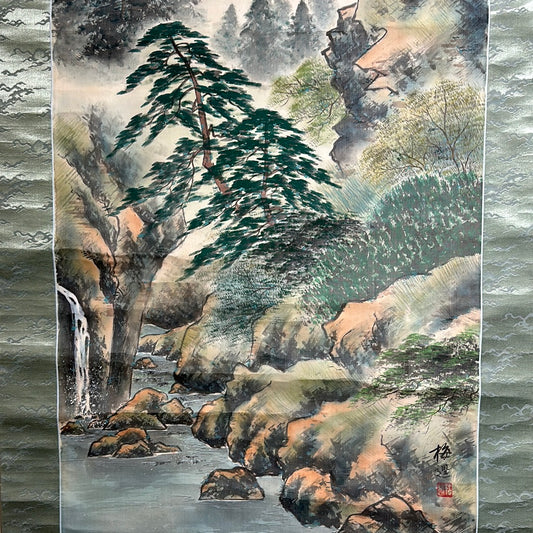The image depicts a piece of Asian artwork affixed to the faux gray siding of an RV. The artwork itself is a delicate, hand-drawn pen and ink watercolor scene characterized by subtle, muted colors. The painting features a picturesque landscape with a small creek and a white waterfall cascading from the center-left, spilling into the river below. Surrounding the river at the bottom left are an assortment of brown and green rocks, adding texture to the scene. 

In the foreground to the right, the rocky terrain rises into a grassy hill, displaying various shades of light and dark green. The intricate details of the grass are meticulously rendered with precise pen strokes. Centered within the image are two leaning pine trees casting shade over the creek, rooted near an overhanging rock. Additional pine trees with sparse foliage appear in the background, partially obscured by distant fog.

Further contributing to the scene's depth are various fine-branched, green trees climbing as high as the image allows. Towards the top right corner, a larger gray mountain laced with fine, lacy green trees rises into the top right side of the artwork. The overall effect is a harmonious blend of nature elements, portraying a tranquil, springtime mountain landscape. Notably, the bottom right corner of the painting features some Asian characters, further emphasizing the artwork's cultural origin.